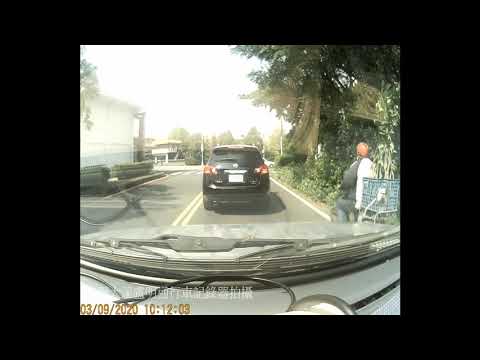This image, captured by a dash cam on March 9, 2020, at 10:12 AM, depicts a sunlit, two-lane road in what appears to be a tropical or warm region, suggested by the presence of palm trees and lush greenery. In the foreground, the dashboard and hood of the recording vehicle are visible, indicating it might be a gray car. Directly ahead, a black SUV is stopped, possibly at a stop sign or traffic light, with more vehicles visible, suggesting an impending intersection turn. To the right, a cyclist with a cube-shaped crate on the back of his bike is also stopped, adding to the scene's dynamic. The cyclist's appearance and various text in either Chinese or Japanese on signs suggest this could be in a Southeast Asian or similar locality. Adjacent to the road are some white, one to two-story buildings, contributing to the urban yet verdant ambiance.